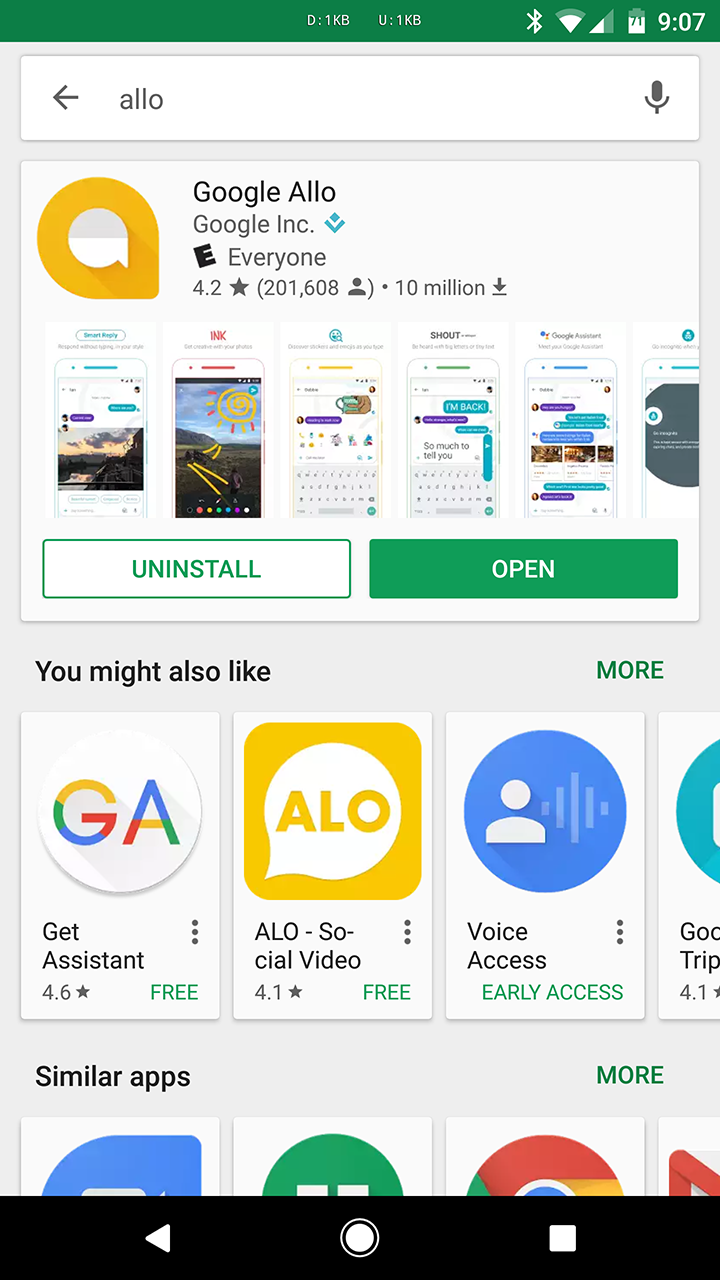A screenshot of the Google Play Store interface is displayed. At the top of the image, there is a search bar with the term "Allo" entered. Below the search bar, the result "Google Allo" is prominently featured, showing a 4.2-star rating based on reviews from 200,608 users. The app has been downloaded over 10 million times, but in this instance, it remains uninstalled. To the right, there is a button labeled "Open." 

Beneath this main section, the interface suggests additional apps with the header "You might also like." Listed here are various applications that include options like "Google Assistant," an early access app named "Allo," "Social Video," and "Voice Access." Below this section, there are labels for similar applications, although the individual app names are not visible. Additionally, there is an option to view more apps, indicated by the label "More" to the side. The overall layout is typical of the Google Play Store, showcasing a mix of app details and recommendations in a user-friendly interface.